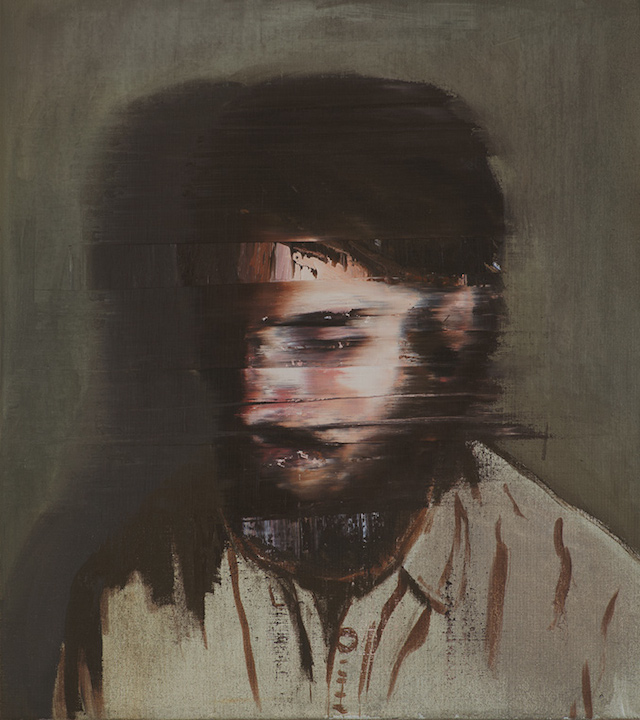The painting vividly portrays a man facing slightly to the left against a gray background. His dark hair, beard, and mustache frame his downcast eyes, conveying a mood of introspection. The artist employs a unique blurring effect that gives the impression of the man glitching, adding a surreal quality to the piece. He is dressed in a pristine white button-down shirt with a neatly folded collar. A shadow, cast to the left, accentuates his presence within the composition. Notably, there is no visible signature from the artist nor any writing on the painting. The scene is minimalistic, devoid of animals, plants, trees, or flowers, focusing entirely on the human figure and his enigmatic aura.